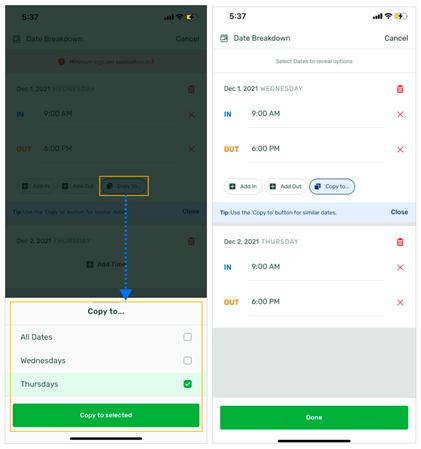**Caption:**

The side-by-side cell phone images depict a scheduling interface with various color-coded elements and detailed information. 

**Left Image:**
- The top portion of the image has a gray film, with an orange box highlighting the "Copy To" button. 
- Within the gray overlay, there's a blue dotted line leading to an arrow pointing somewhere on the screen. 
- The bottom of the image also features an orange box around another "Copy To" button. 
- The main section displays weekdays, with Wednesday and Thursday visible. Thursday appears to be selected.
- Below this, there's a green button labeled "Copy to Selected."

**Right Image:**
- The right image offers a breakdown of dates and times.
- It starts with a "Cancel" option followed by a detailed schedule for December 1, 2021.
  - The schedule reads: Wednesday, 9 a.m. - 6 p.m., with options to "Add In" and "Add Out" next to "Copy To" buttons, highlighted in blue.
- A blue banner at the bottom provides a tip: "Use the 'Copy To' button for similar dates."
- Below the banner, the schedule continues with December 2, 2021, for Thursday, showing the same time frame (9 a.m. - 6 p.m.).
  - Red check marks indicate the 'In' and 'Out' times, and a red garbage can icon is present above the date.

The images use a variety of colors, including gray, orange, blue, green, black, white, and red, to differentiate various elements and actions in the scheduling interface.